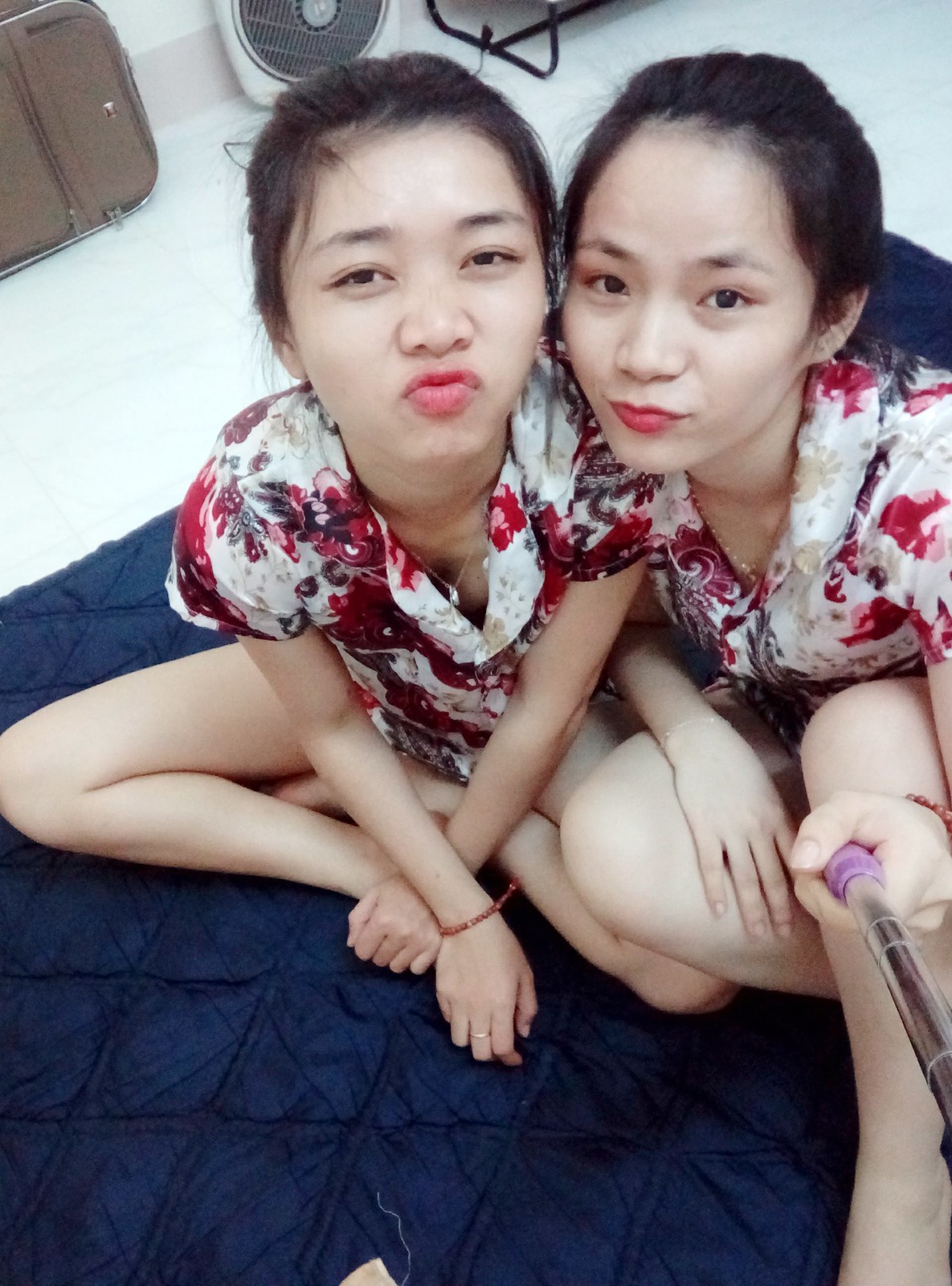The image captures an indoor setting featuring two young Asian women with dark hair pulled back into ponytails. They are seated on a dark blue carpet or rug, and appear to be taking a selfie together. The woman on the right, who is holding a selfie stick with a purple handle and silver stick, is clad in a white dress or a white shirt adorned with red flowers. Sitting cross-legged next to her is another woman who is barefoot and has her lips puckered as if ready to kiss. Both women have pale skin, dark eyes, and lipstick, highlighting their pink lips. They're wearing floral shirts with lace collars, accompanied by necklaces and red bracelets. The background showcases a white floor, a white fan, a piece of luggage, and a metal rail or stand. The image is purely photographic with no text.